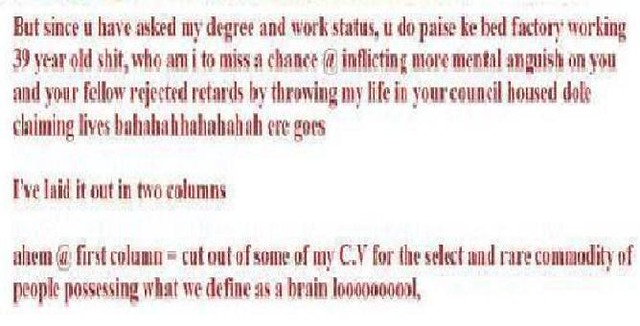This image captures a blurry piece of text in dark red font. Despite the blurriness, it is possible to make out the message, which is riddled with grammatical errors, misspellings, and offensive language. The text reads:

"But you have asked my degree and work status. You do ... factory working 39 year old s-h-i-t. Who am I to miss a chance at inflicting more mental anguish on you and your fellow rejected retards by throwing my life in your council housed dole claiming lives ba ha ha ha ha."

The author sarcastically follows with:

"I've laid it out in two columns. First column: cut out of some of my CV for this select and rare commodity of people possessing what we define as a brain L-O-O-O-O-O-L."

This text is clearly meant to convey a mocking and derogatory tone, highlighting the author’s disdain for an unspecified audience. The image provides a glimpse into the dark and cynical humor of the person who wrote it.